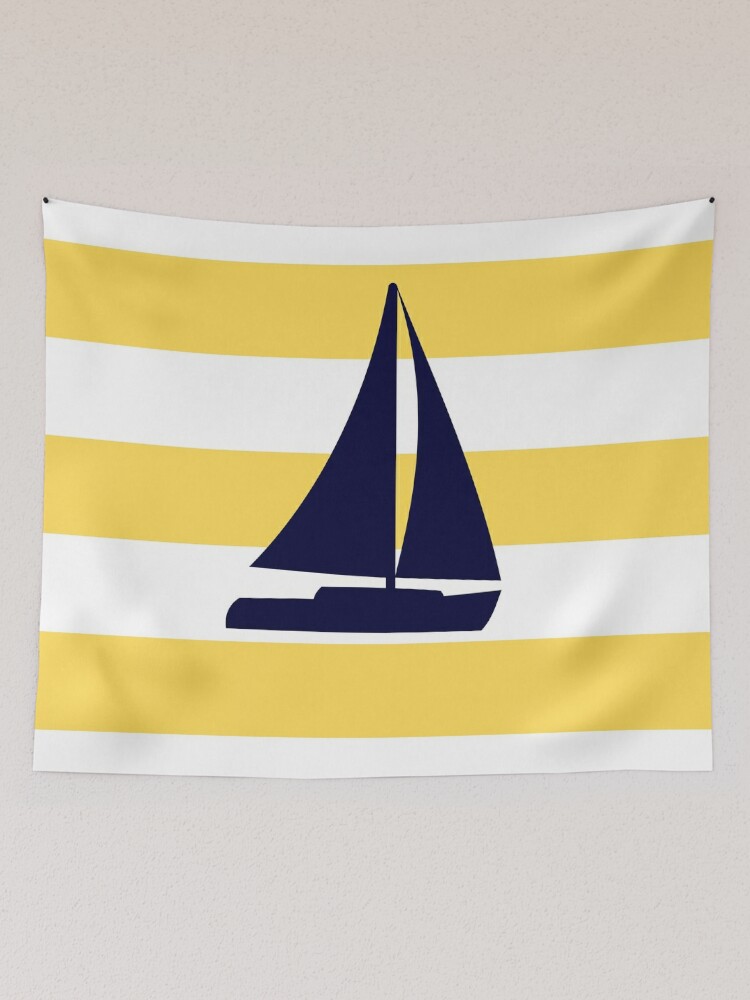This photograph features a simplistic yet striking composition. A square piece of fabric, likely about a foot by a foot in size, is suspended on a white wall, secured by thumbtacks in both the upper left and upper right corners. The fabric itself showcases an alternating pattern of three horizontal yellow bars interspersed with four horizontal white bars, each approximately two inches thick. The focal point of the fabric is a navy blue silhouette of a small, two-masted sailboat sailing towards the right. The boat's design is minimalistic, with a billowed front sail suggestive of movement, as if catching the wind. The mast and sails allow the background stripes to peek through, further highlighting the sailboat's silhouette against the simple yet vivid backdrop.